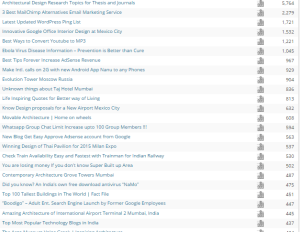The image features a significant amount of low-resolution text, making it difficult to read. The text is displayed in a turquoise color that contributes to its poor legibility. There are approximately 24 and a half lines of this text. An icon is present on the right side of the image, though its details are indiscernible. Each line of text is accompanied by a number, starting from the top with some lines hinting at topics like "Advanced Design Research." Another discernible text includes the word “services” with a number, 2,279, next to it. The text is presented in a teal blue color, with alternating gray and white backgrounds, and the numbers appear to be in gray. There seems to be no black text or elements in the image.